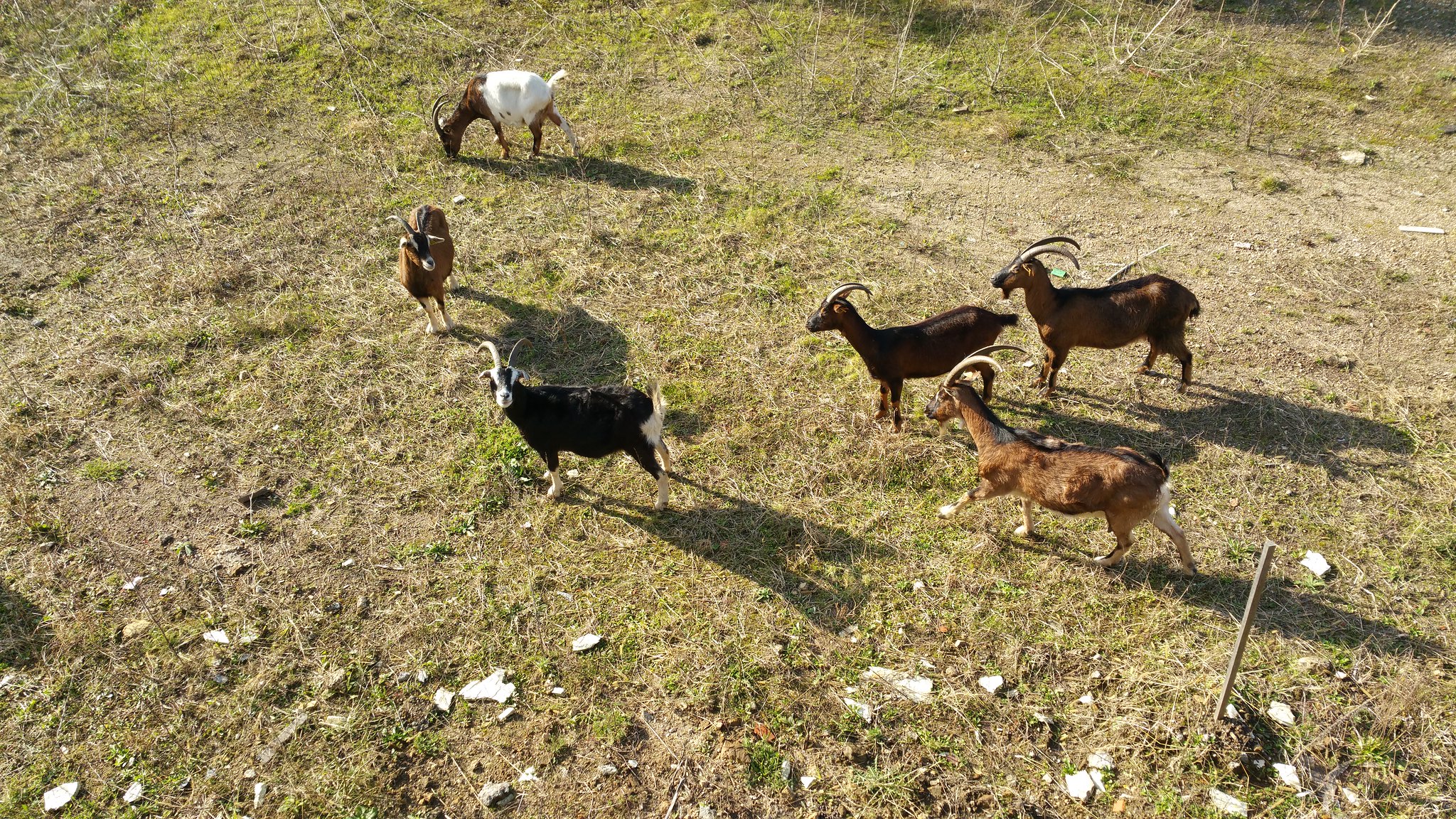In this vivid outdoor photograph, a picturesque grassy meadow stretches beneath a bright blue sky. The grassland, peppered with patches of greyish-brown dirt and rocks, creates a rustic ambiance. Centered in the scene are six male goats, each adorned with long, curling horns. The focus is drawn to a white and brown goat busily grazing on the verdant grass. Beside him is a brown goat with a lighter snout, casually observing the surroundings. Moving to the front, a black goat with a white tush, tail, and facial markings gazes directly at the camera, his body oriented to the left. In the background, two more goats, both black, look off to the left, while a brown goat below them appears to be trotting towards the pair. The day seems pleasant, as evidenced by the soft shadows cast by the goats onto the grass, hinting at the sun's high position in the sky. Adding to the pastoral charm, a wooden post visible in the distance suggests the possible boundary of a ranch or a corral.